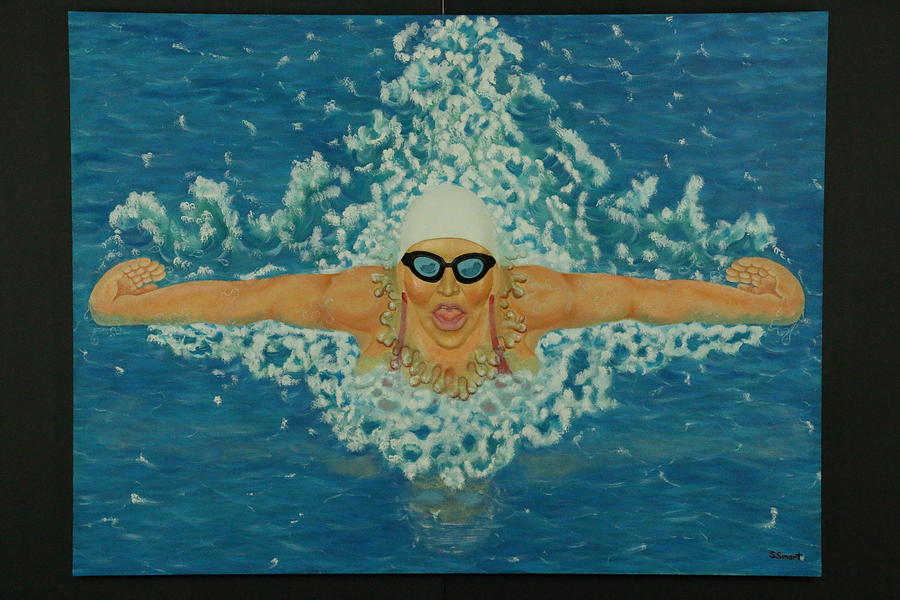The image is a detailed digital cartoon illustration depicting a female swimmer in a vibrant blue pool. The landscape-oriented image is framed by an uneven black border, thicker on the sides than the top and bottom. The swimmer, viewed face-on, is breaching the surface of the water, creating foam shaped almost like her body. The water around her is dark blue with slight white peaks and swirls, indicating motion.

The swimmer appears to be an older woman, wearing a white swim cap, black-rimmed goggles with blue lenses, and a potentially pink bathing suit limitedly visible via the shoulder straps. Her mouth is open with her tongue slightly exposed. Both her arms are stretched outwards along the horizon, hands curled inwards at a 45-degree angle behind her. She leaves white, almost worm-like, ripples in the water behind her, rendering the scene dynamic and lively. The illustration captures her moment of breaststroke, suggested by her arm and hand positioning.